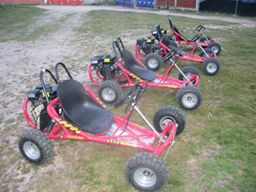In this detailed photograph, we see four red go-karts lined up side by side on a patchy lawn. The lawn is uneven, with green grass on the right side, giving way to bare dirt and rockier ground on the left. Each go-kart has a single, curved black plastic seat and is built with a red framed tube steel structure. These go-karts are equipped with knobby, all-terrain wheels attached via silver metal hubs, and they have black lawnmower engines mounted at the back. The steering wheel is centrally positioned near the front axle, supported by additional red bars. There's an M-shaped roll bar behind the seat, adorned with yellow and black caution stripes, likely providing minimal protection to the driver and engine. In the background, a dirt path leads up to a building with a red base and hints of blue color, and a red gate or fence can be seen vaguely outlining part of the area.